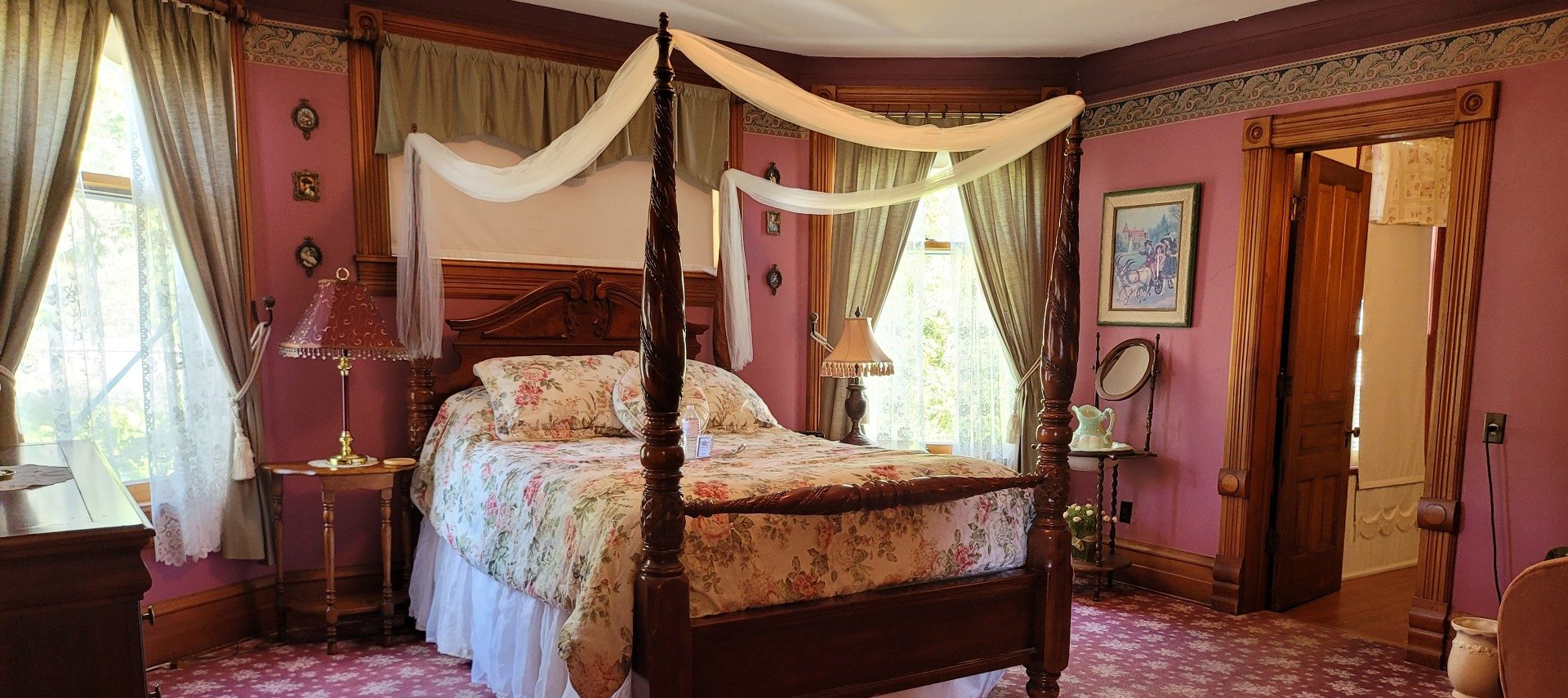The image depicts a vintage 1920s or 30s style bedroom, likely in a hotel or Airbnb. The focal point is a large, imposing four-poster bed with dark, spiral-carved wooden posts that nearly reach the ceiling. The bed is adorned with a cream-colored duvet featuring a pink and green floral pattern, complemented by a white bed skirt and two pillows. A delicate white mosquito netting drapes across the top of the bed.

The room's walls are painted a rosy pink with a reddish-brown border near the white ceiling. Pink floral patterned carpet covers the floor. There are tall windows on each side of the bed, framed with dark wooden frames and dressed in dark gray-green drapes that are tied back with white ropes, revealing a second layer of delicate, patterned white curtains underneath.

Flanking the bed are small wooden tables each with a lamp; the left one boasts a dark burgundy velvet lampshade, while the right one has a beige-white shade with fringed detailing. To the right of the bedroom is a washstand featuring a white ceramic pitcher and a piece of framed art above it. This washstand is positioned against a pink wall, matching the overall color scheme, and a door on the right side of the room leads to an adjacent bathroom. The overall style of the photograph captures a sense of photographic representationalism realism, emphasizing the period charm and careful detailing of the decor.